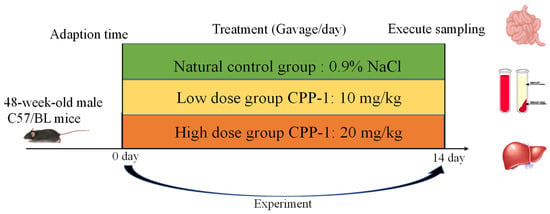The image appears to be an infographic extracted from a scientific textbook, detailing an experiment involving 48-week-old male C57-BL mice. The setup spans from 0 to 14 days and is divided into adaptation time, treatment, gavage per day, and execute sampling phases. Three color-coded groups are depicted in a three-row box: the top row is green representing the natural control group with 0.9% NaCl, the middle row is yellow for the low dose group administered CPP-1 at 10 mg/kg, and the bottom row is orange for the high dose group administered CPP-1 at 20 mg/kg. An arrow at the bottom highlights that the experiment lasts for 14 days. On the right side, there are additional graphics including a brain, test tubes with varying contents, and lungs, adding visual context to the infographic.